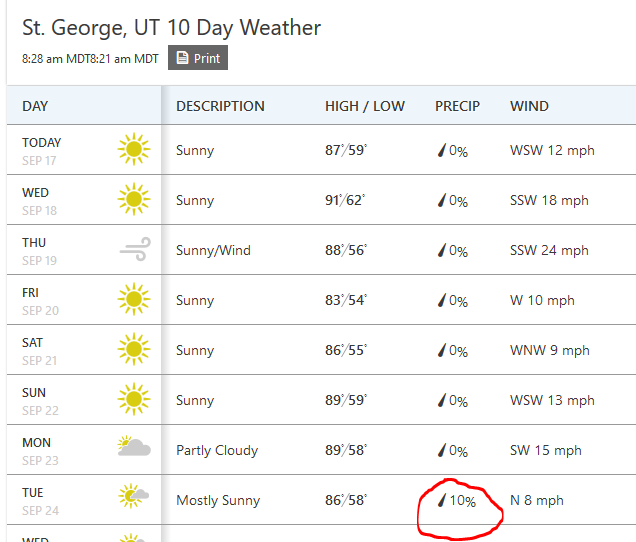In the top left corner of the image, there's text indicating "St. George, UT", with "UT" capitalized. It also mentions a "10-day weather forecast". Below this header, the current time is displayed as "8:28 a.m." next to "MDT", and again "8:21 a.m." with "MDT". Positioned nearby is a black rectangle featuring the word "print" and an icon of a piece of paper.

On the left side, there is a blue rectangle labeled "day", followed by today's date, "September 17th". An icon of a sun accompanied by the description "sunny" details today's weather forecast. The predicted high is 87°F, with a low of 59°F, 0% chance of precipitation, and winds from the WSW at 12 miles per hour.

Moving to Thursday, September 19th, the forecast changes slightly, displaying a sunny and windy day. The high is expected to reach 88°F, with a low of 56°F, 0% chance of precipitation, and southwest winds blowing at 24 miles per hour.

The forecast for Friday, Saturday, and Sunday indicates sunny weather for all three days. On Monday, the weather shifts to partly cloudy, with a high of 89°F, a low of 58°F, zero precipitation, and southwest winds at 15 miles per hour.

Finally, at the bottom of the image, Tuesday, September 24th, is described as a mostly sunny day. A section circled in red highlights the precipitation, depicted by a gray raindrop icon with a 10% chance for rain.